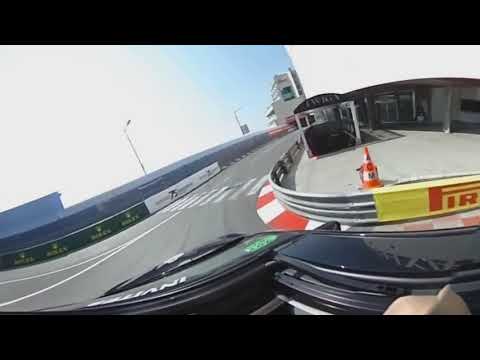This detailed photograph, taken from the perspective of someone driving a race car, showcases a scene on what appears to be a racetrack or closed city street circuit. Dominating the bottom right corner of the image is the car's black hood, emblazoned with partially visible white letters ending in "A-N-I." The vehicle is navigating a sharp right-hand turn, with the road curving towards the center of the frame and bordered by metal guardrails to prevent collision with nearby structures. The scene is set in an urban environment, evidenced by a pedestrian crosswalk, streetlights, and a white building in the top left corner. A prominent Pirelli tire advertisement is visible at the curve, along with a pylon marked "AM." This race track setting, enhanced by these details, is seemingly near an ocean, adding a layer of scenic backdrop to the intense racing atmosphere.